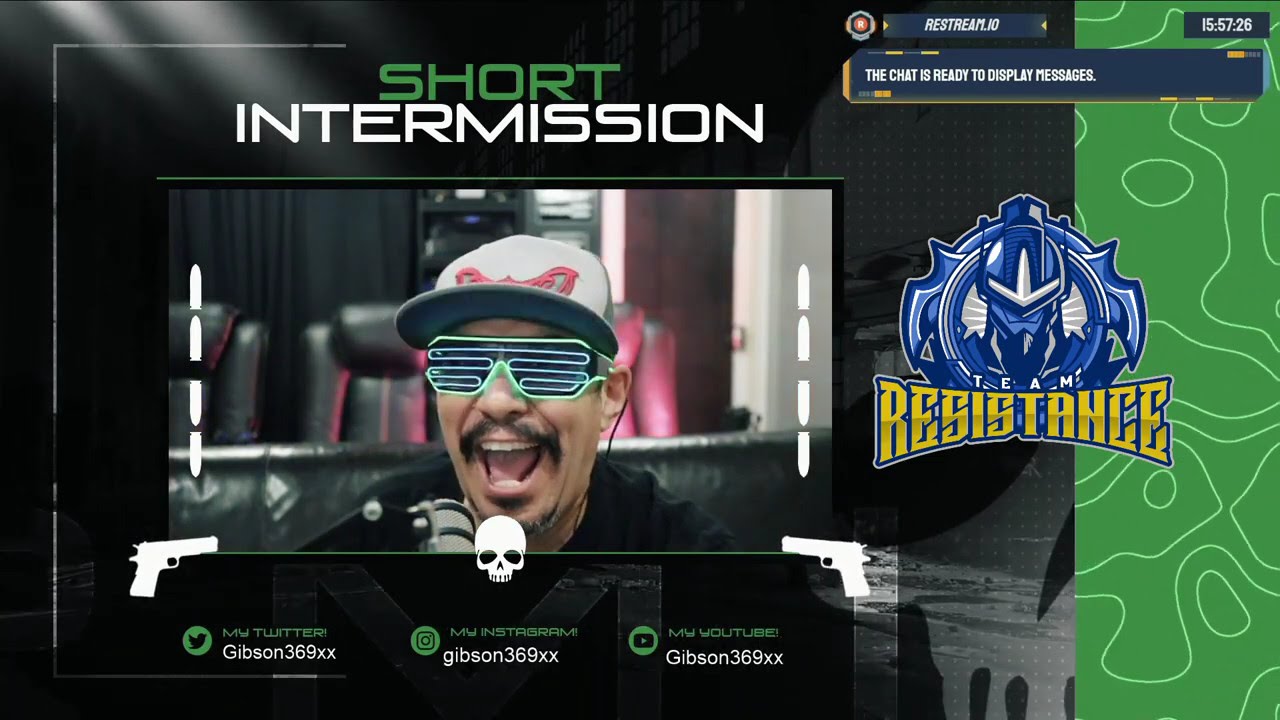In this screenshot from a gaming environment, a man is featured at the center, wearing stylized, neon green sunglasses with horizontal fluorescent green lines. His expression is one of excitement, mouth open wide, revealing a playful demeanor. He sports a goatee and a baseball cap with a blue rim, a white top, and red lettering. Above the man’s image, the text "Short Intermission" is displayed, with "Short" in green and "Intermission" in white. Below his chin, a skull flanked by the white silhouettes of two guns is visible. Beneath these images, the text "Gibson 369 XX" is prominently displayed, followed by potential social media tags such as Twitter, Instagram, and YouTube, though their exact abbreviations are unclear. To the left of this central image, there is a small logo featuring a robot and the words "Team Resistance" in blue. In the top area of the screen, additional details such as "RestStream.no 15:57:26" and "The chat is ready to display messages" are noted, suggesting that this is part of a live stream or an online game interface. A microphone is visible in front of the man, affirming the interactive, broadcast nature of the scene.